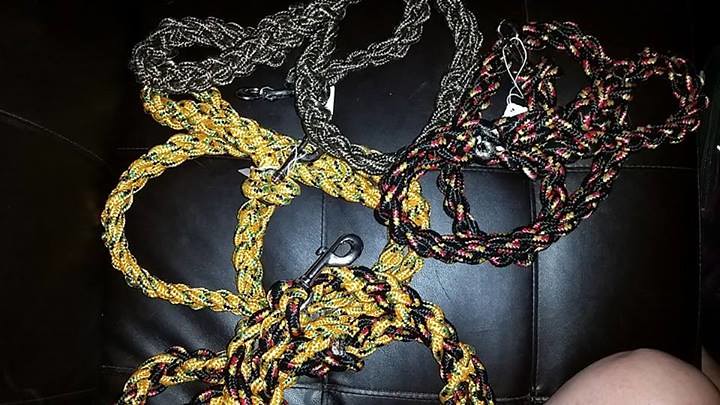The photograph captures a set of four dog leashes meticulously arranged on a black leather ottoman or cushion. Each leash features a distinct braided design and color pattern. The first leash, positioned towards the top, is predominantly silvery gray with a metallic clip at the end. Directly below it, a second leash displays a more vibrant palette of yellow, black, orange, and silver. To the right, a third leash combines yellow, black, and red hues, also equipped with a silver clip. The fourth leash, resting below the others, melds shades of black, red, yellow, and a touch of orange, intertwining slightly with the other leashes. These leashes, each terminating in a functional, metal clasp designed to attach securely to a dog’s collar, create a visually complex arrangement. In the lower right corner, a portion of a person’s knee subtly enters the frame, adding a touch of human presence to the image.